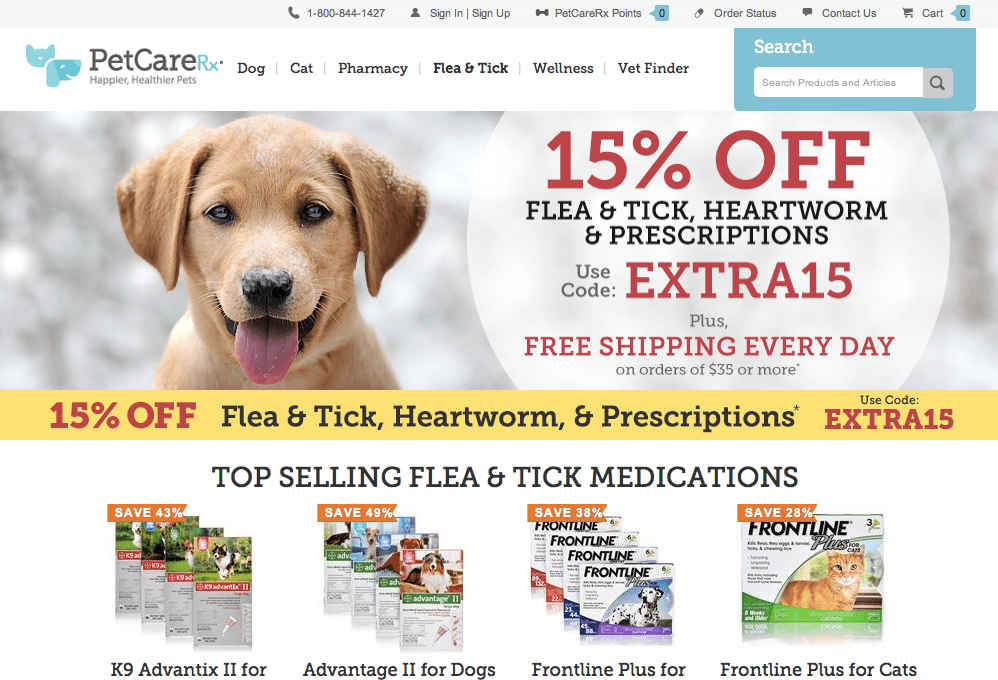**PetCare Rx Website UI Description**

The website interface for PetCare Rx, also known as PetCare Prescriptions, features a clean, structured design with a focus on pet medications and care products. At the top of the site, there's a header bar containing essential navigational and contact information. This bar includes a phone icon followed by the customer service number, 1-800-844-1427. To the right, there's an icon of a person with options to "Sign In" and "Sign Up," separated by a vertical line. Additionally, there's a dog bone icon indicating "PetCare Rx Points" with a speech bubble highlighting the point system. Further along, there's an "Order Status" button, represented by a pill icon, a "Contact Us" button with a speech bubble icon, and a shopping cart icon showing the cart status as empty, all set against an aqua-colored background.

To the left of the header, the website's logo is prominently displayed within a light gray box. This logo includes an outline of a cat and a dog in aqua color, with "PetCare" written in gray, a blue "Rx," and the tagline "Happier, Healthier Pets." Below the logo, the main navigation menu includes categories such as Dog, Cat, Pharmacy, Flea and Tick, Wellness, and Vet Finder, each separated by a vertical line.

A search box with an aqua-blue background is present below the navigation menu, allowing users to search for products and articles. The search box contains white text and a magnifying glass icon inside a light gray square.

The main content area of the site features a visually appealing image of a light brown puppy with snow on its nose, head, and ears, set against a snowy background with trees. The cute puppy has brown eyes and is depicted with a playful expression, tongue out, and appears to be smiling. Superimposed over the image is a white, partially cut-off circle that reads "15% off" in red text, along with "Flea and Tick, Heartworm, and Prescriptions" in black text. Additionally, it mentions "Use code" in black text followed by "EXTRA 15" in red text, and notes "Plus free shipping every day on orders of $35 or more" in gray text.

Below this promotional banner, there's a yellow rectangle with similar promotional text, reiterating the "15% off" for flea and tick, heartworm, and prescription products using code "EXTRA 15."

Following this, the site showcases a series of product images with discount banners. The first product features a "Save 43%" banner in white text on an orange background and displays four staggered boxes of Canine Advantix II, suggesting it's intended for dogs. The second product, with a "Save 49%" banner, showcases Advantix II for dogs with similar staggered image boxes. Another product shows a "Save 38%" banner for Frontline Plus, also featuring images of dogs, while the last product highlights Frontline Plus for cats with a tabby cat image and a "Save 28%" banner. This section is titled "Top-selling Flea and Tick Medications."

Overall, the PetCare Rx website is clearly designed to provide detailed information and offers on pet medications and care products, ensuring a user-friendly experience for pet owners seeking reliable healthcare solutions for their pets.